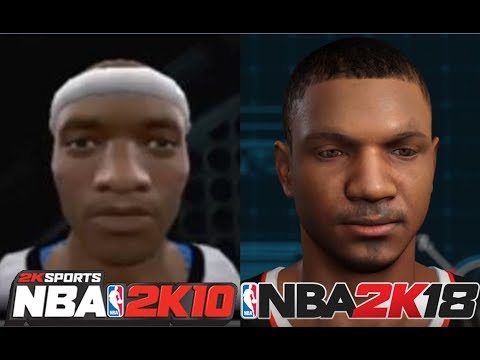Here are side-by-side images comparing the graphics of NBA2K10 and NBA2K18, showcasing a clear evolution in visual fidelity over the years. Both images display the same, potentially custom, in-game player rendering. On the left, in NBA2K10, the player's face appears markedly pixelated with low texture detail, giving it a simple and less realistic look. The facial features, like the hairline and eyebrows, lack sharpness and definition, epitomizing the graphical limitations of that era. Contrastingly, the right image, representing NBA2K18, reveals a dramatic improvement in graphical quality. The player's face is rendered with high attention to detail, with noticeable textures on the skin, well-defined hairline, and realistic facial hair, making it appear almost lifelike. This comparison vividly illustrates the generational leaps in video game graphics, highlighting the advancements made over eight years.